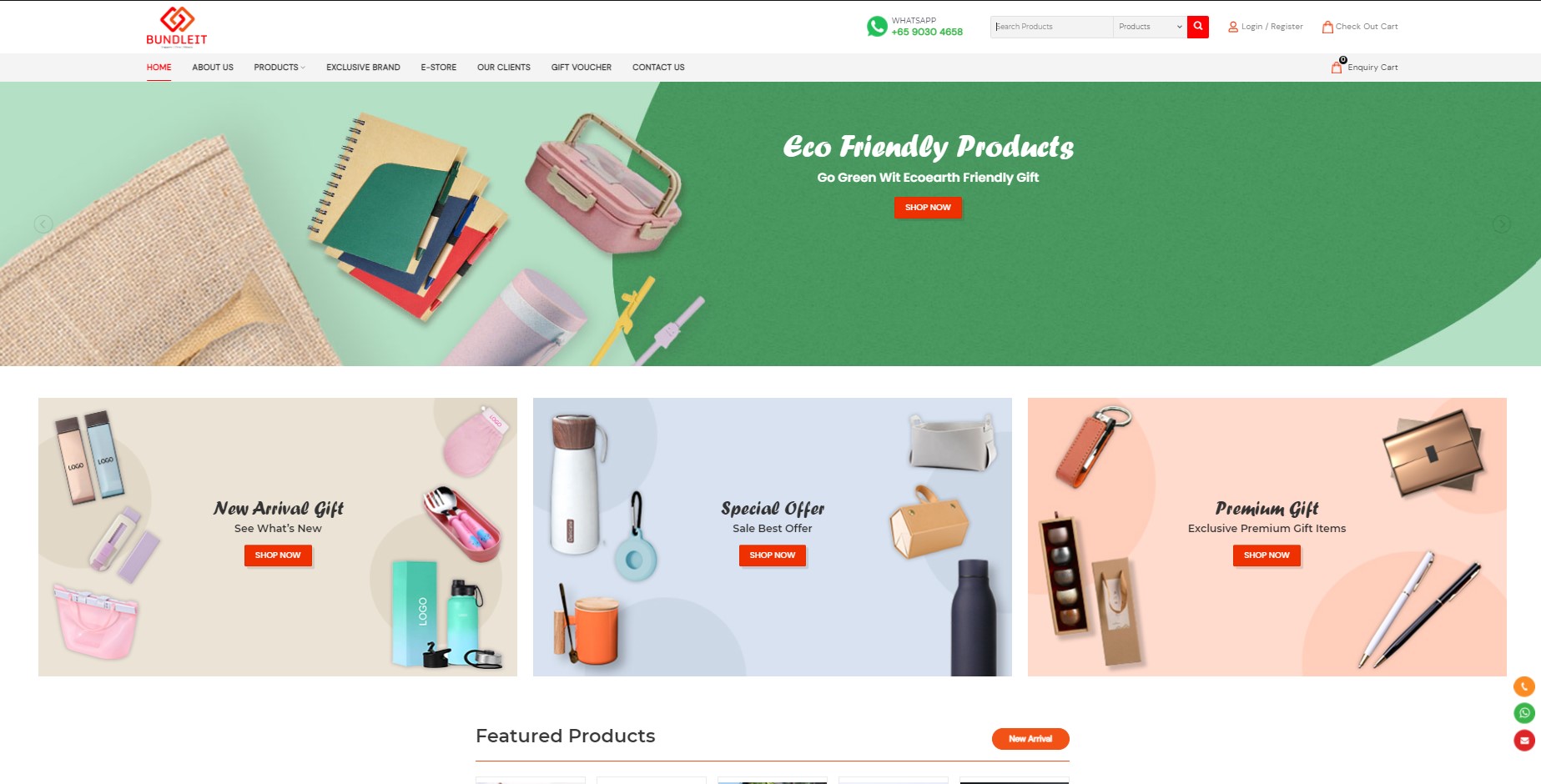The image is a detailed screenshot of the Bundlet website. In the upper left corner, the Bundlet logo is prominently displayed, featuring two interlocked red squares or diamonds and the word "BUNDLET" in bold, red uppercase letters. To the upper right, the "Log In" and "Register" options are clearly visible, allowing users to access their accounts or sign up.

Just below, a horizontal navigation menu offers links to various sections of the website: Home, About Us, Products, Exclusive Brand, E-Store, Our Clients, Gift Voucher, and Contact Us. Dominating the center of the screen is a large, eye-catching image spanning the full width, showcasing an array of eco-friendly supplies. Superimposed on this image in white text, the phrases "Eco-friendly Products," "Go Green with Eco-worth," and "Friendly Gift" are prominently displayed, accompanied by a striking red call-to-action button labeled "Shop Now."

Below the large image, the webpage is divided into three distinct sections. On the left, a section titled "New Arrival Gift" invites visitors to "See What's New" with a corresponding "Shop Now" button, urging them to explore the latest additions. The center section highlights a "Special Offer," enticing customers with "Sale Best Offer" and another "Shop Now" button for immediate action. The right section focuses on "Premium Gift" items, promoting "Exclusive Premium Gift Items" and featuring a similar red "Shop Now" button to encourage further browsing.